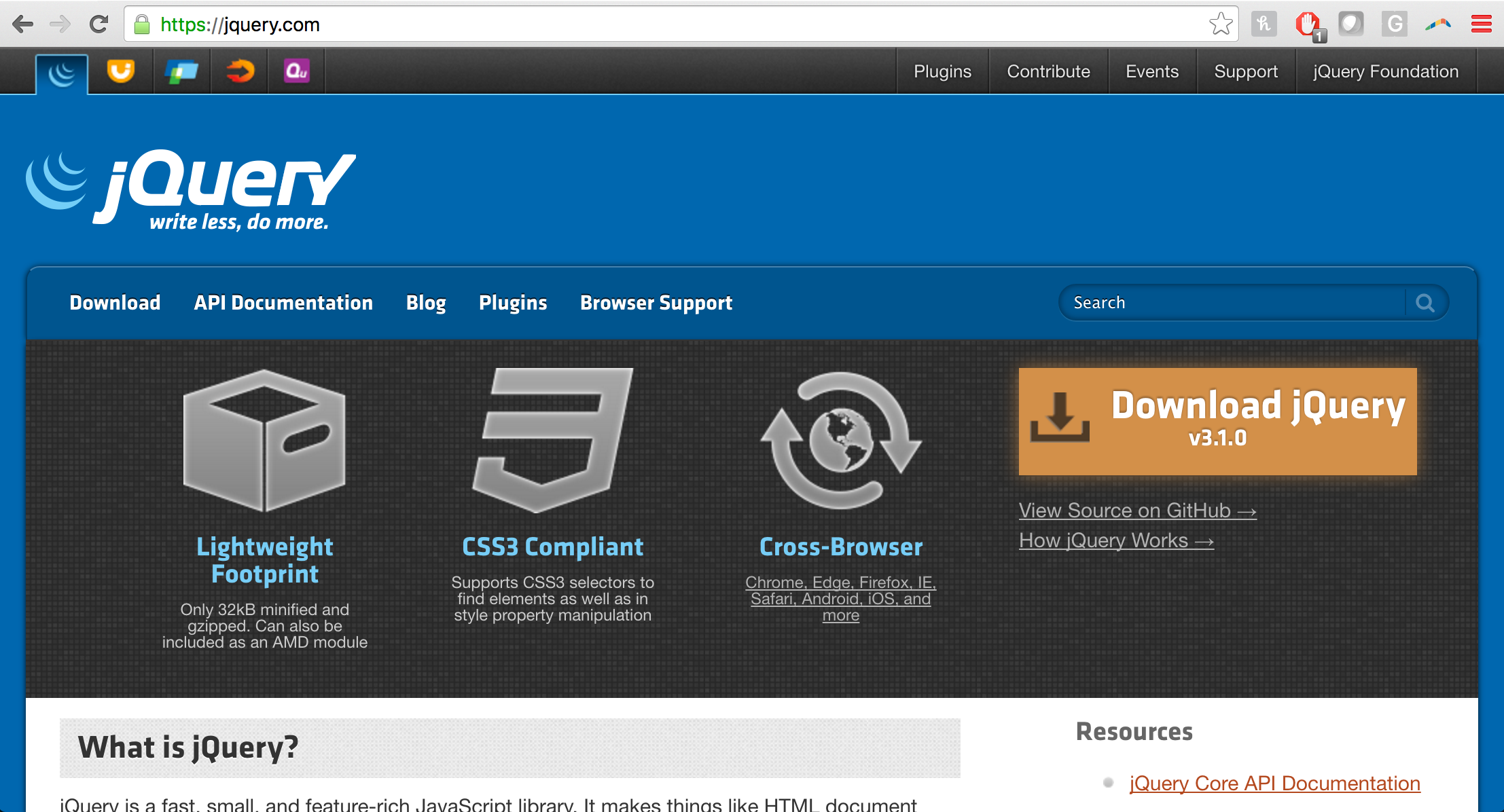The homepage of the jQuery website features a sleek, modern design with a predominantly dark theme. At the top of the page, there's a prominent black navigation bar with links to "Plugins," "Contribute," "Events," "Support," and the "jQuery Foundation." Below this, a light blue box prominently displays the jQuery slogan, "Write Less, Do More." Beneath this banner, a darker blue box offers quick links to essential resources such as "Download," "API Documentation," "Blog," "Plugins," and "Browser Support." To the far right of this box, there's a search function for easy navigation.

Against the black background, there's an informative section titled "Lightweight Footprint." This section highlights an image of a box and mentions that jQuery is just 32 KB when minified and gzipped. It also emphasizes that it can be integrated as an AMD module, is CS53 compliant, and works seamlessly across various browsers including Chrome, Edge, Firefox, Safari, as well as on Android and iOS devices.

An orange call-to-action button labeled "Download jQuery" appears prominently, followed by links to "View Source on GitHub" and "How jQuery Works." Underneath the aforementioned sections is a heading, "What is jQuery?" which invites users to learn more about the platform's functionalities and benefits.